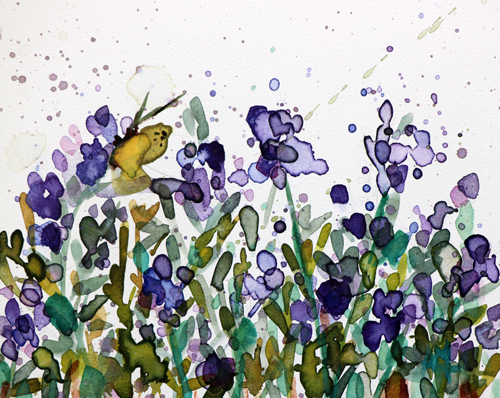This is a square, watercolor painting of a field of flowers with no border. The background is predominantly white, with splashes of paint, mostly purple, scattered throughout. The flowers, depicted in various shades of purple, don't all conform to typical floral shapes, lending an abstract and splotchy appearance to the artwork. Green and brown hues are used for the stems and leaves, adding depth and variation in color. On the left middle area of the painting, there appears to be a small yellow butterfly with a black body and long black antenna, perched delicately on one of the flowers. The top portion of the painting, representing the sky, is left blank, except for a scattering of colored circles that might symbolize pollen. The entire image has a blurred, expressionistic quality, typical of watercolor technique, and does not contain any text or signature.